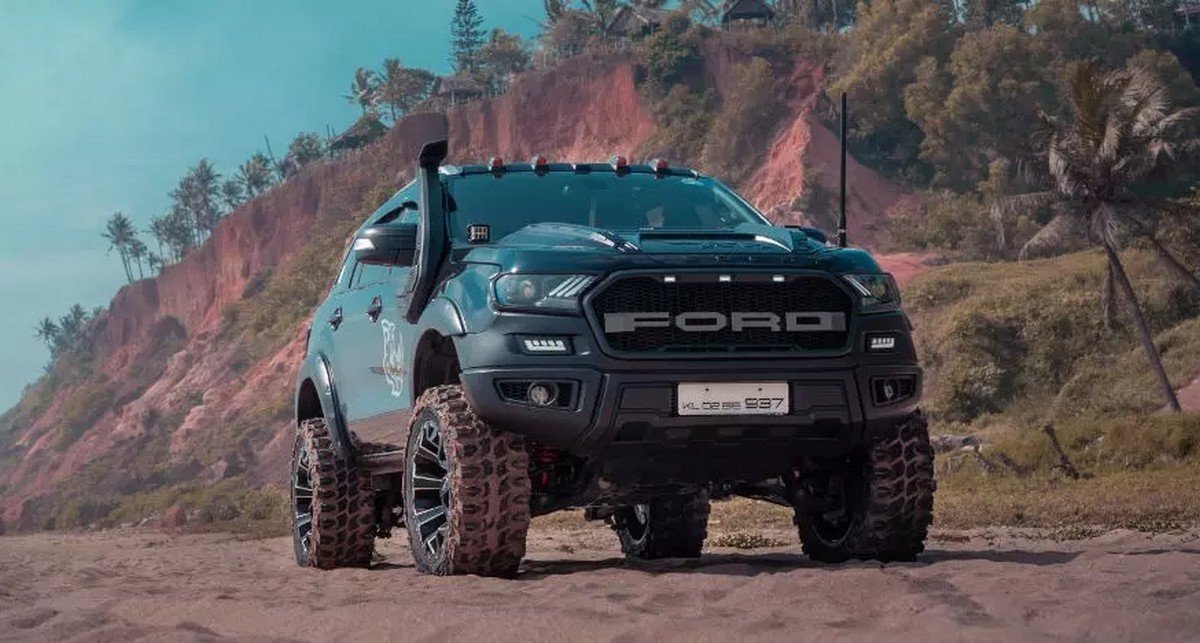The image captures a rugged outdoor scene dominated by a customized, dark green Ford Ranger or similar mid-sized pickup truck, outfitted for off-road adventures. The truck features super large off-road tires, a lifted suspension system, and a black brush guard on the front bumper. Atop the vehicle is a roof rack with a light bar, alongside noticeable white fender flares and a snorkel on the driver's side. The front of the truck prominently displays the Ford logo and a white license plate below it. The vehicle's windows are small, adding to its tank-like appearance. 

The scene unfolds against a backdrop of scenic natural elements, with rocky cliffs showing signs of erosion and dotted with trees and shrubs, including palm trees, under a clear blue sky with wispy white clouds. The foreground reveals a sandy, dirt-laden terrain that complements the rugged, adventurous spirit of the truck. The main focus of the image is the off-roading vehicle, facing slightly off-center to the left, perfectly embodying a blend of adventure and wilderness.